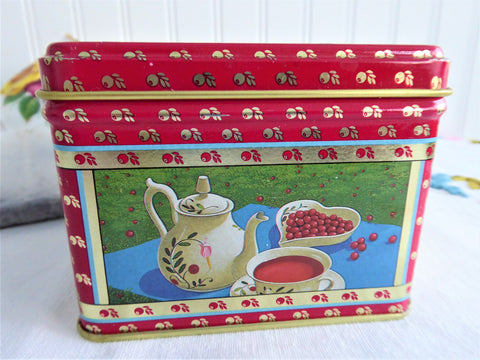This close-up image depicts a red, metal tin resembling a teabox. It's slightly tilted, with its right side closer to the viewer in perspective. The tin rests on a white surface, which casts subtle shadows, and is backed by a wall featuring white panel tiles. The tin itself is adorned with gold emblems and has intricate red and gold markings on the top and bottom sections. At the center of the tin, there's an elaborate, framed image featuring a white ceramic teapot, a teacup on a saucer, and a harp-shaped bowl filled with what appear to be cranberries or cherries. The teacup, decorated with floral designs, contains a light red liquid. The framed image has tan and light blue borders, contrasting with the dominant red color of the tin. There is no text visible on the tin, and the overall quality of the image is quite high, capturing fine details and subtle shadows.